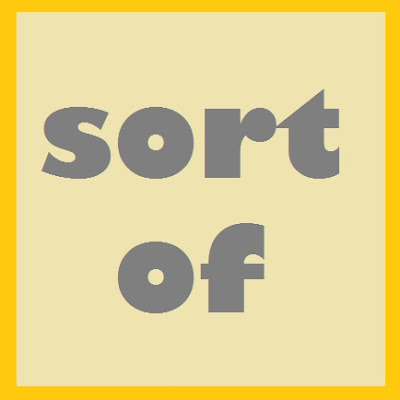The image features a nearly square rectangle with a deep yellow border. The background inside the rectangle is a faded pink hue. In the middle of this rectangle, in large, playful lowercase font, the phrase "sort of" is written in a bold gray color. The text is carefully centered, both horizontally and vertically, creating a balanced and neat appearance. The deep yellow outline contrasts with the light background, emphasizing the central playful yet indecisive text, which gives the entire image a humorous tone.